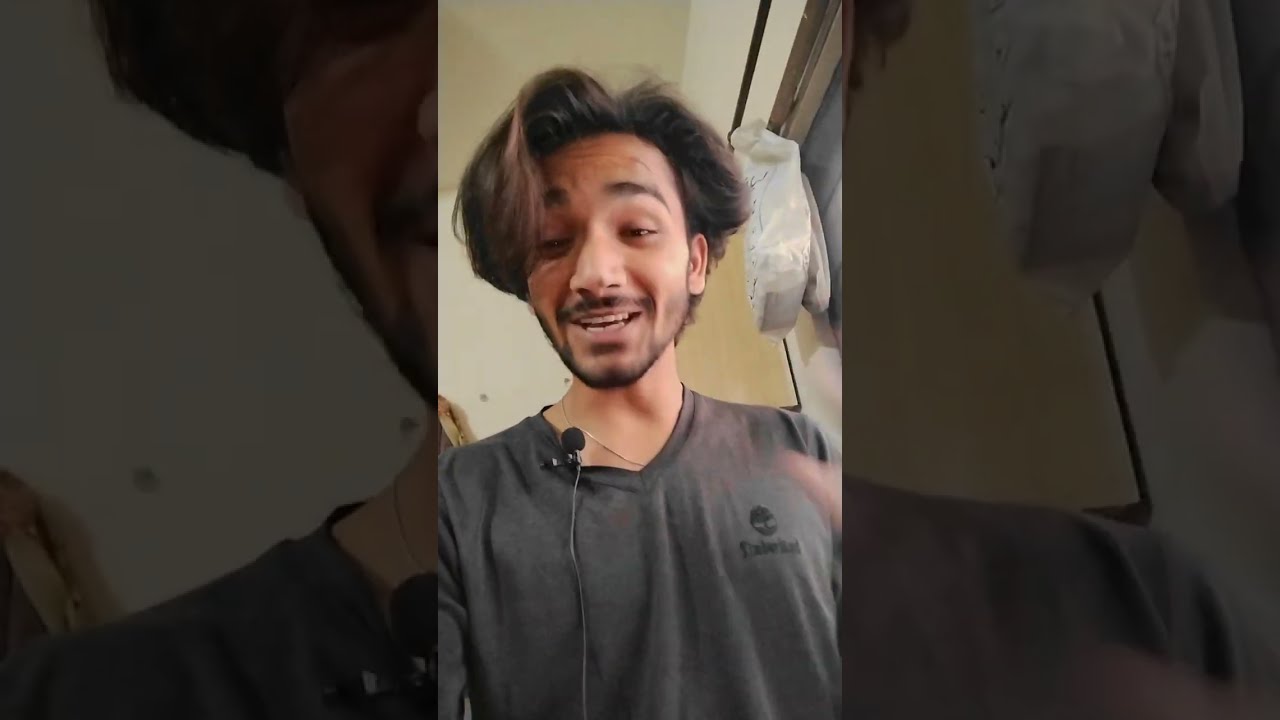The image features a horizontally rectangular, three-panel composition with the central panel being the smallest. It depicts a young man indoors, highlighted in color. The middle panel showcases him in focus, wearing a gray long-sleeved T-shirt with an unreadable logo. Affixed to the collar of his shirt is a microphone, with the wire running down the right side of his chest. He also wears a gold chain around his neck. His facial hair consists of a goatee and a light mustache, and his hair is dark brown with possible highlights, styled and slightly falling into his face. The man appears to be speaking into the microphone, his mouth slightly open, and is looking downwards, as if towards a camera, possibly engaged in a selfie video or a virtual meeting. Behind him is a yellowish wall with black trim and an indistinguishable object hanging to his right.